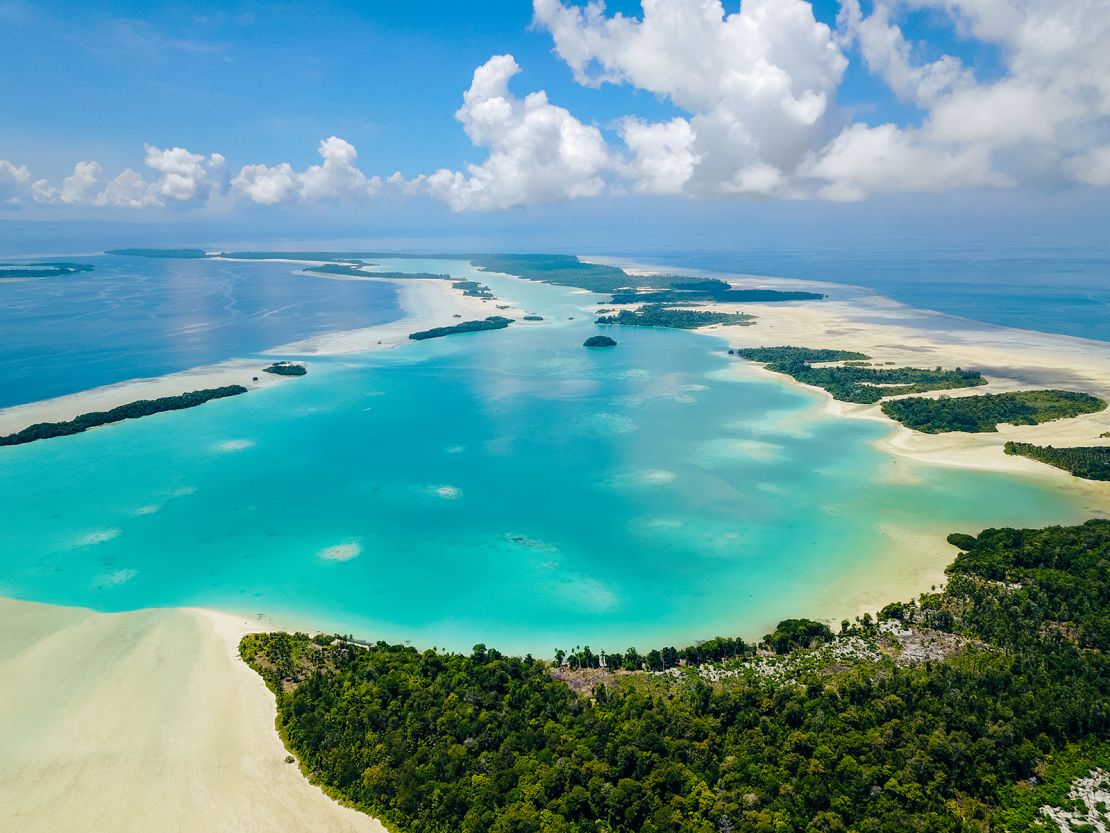This detailed drone photograph captures an expansive, vibrant Caribbean seascape bathed in sunlight. The image, taken from above in landscape orientation, showcases a stunning blend of aquatic and terrestrial elements. In the foreground, the bay's crystal-clear, aqua-colored water transitions seamlessly to the deeper, darker blue of the ocean, reflecting the bright blue sky adorned with puffy white clouds.

The lower half of the image features a sweeping curved landmass. On the left, a pristine white sandy beach meets the shoreline, bordered by lush green trees creating a vivid contrast. To the right, the greenery is denser, comprising primarily deciduous trees. Nestled near the top of the curve is a small section housing some structures, hinting at human presence amidst the natural beauty.

The coastline continues around the right side of the frame and recedes toward the horizon, encapsulating the serene essence of the water meeting the land. An additional strip of sandy beach extends from the center left, pointing towards the main curve, enhancing the depth and layers within the composition. The entire scene evokes a sense of tranquility and untouched paradise, typical of Caribbean islands, captured in exquisite photographic realism.